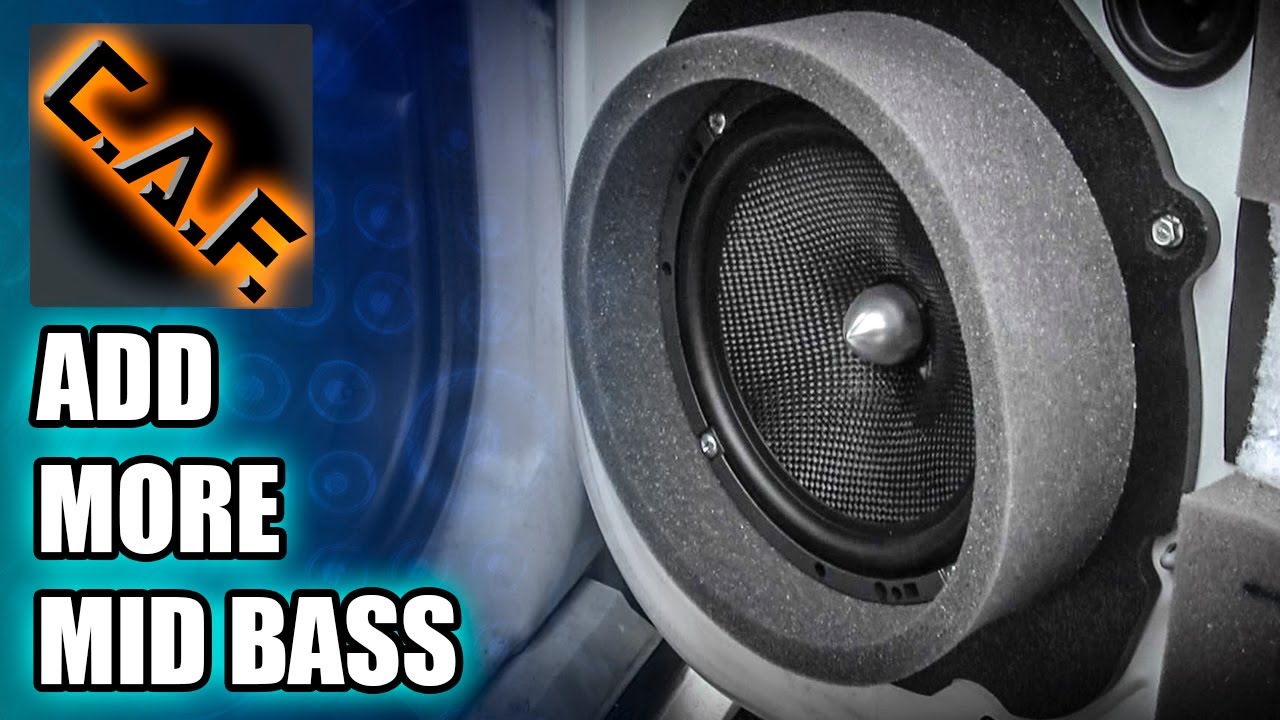The image is a detailed, black and white close-up of a powerful-looking bass speaker, typically integrated into a car's sound system. The front of the speaker prominently displays its solid and compact construction, revealing the intricacies of the mesh and surrounding foam. On the top left corner, a black square with black font illuminated by a yellow hue reads "C.A.F." Below that, in white font, it states "add more mid-bass." This image likely serves as a promotional thumbnail for a YouTube video from the CAF channel, offering tips on enhancing mid-bass performance in car audio systems.